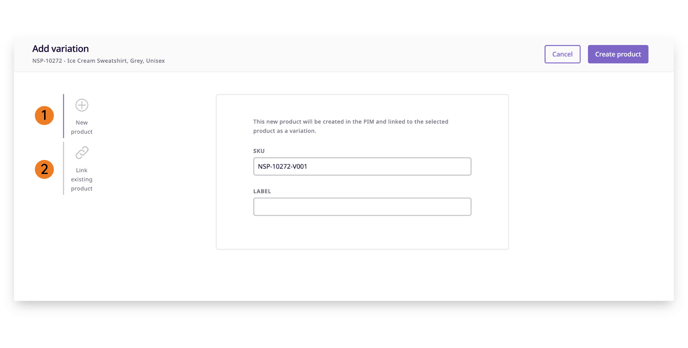The image features a detailed layout of a product management interface. The background at the top is grey, overlaid with black text that reads "Add Variation." Below this header, grey text displays "NSP-272 Ice Cream Sweatshirt Grey Unisex."

On the right-hand side, two buttons are present: a white button with blue text that says "Cancel," and a blue button with white text labeled "Create Production."

On the left side of the white background, there are various circular icons. The first icon is a yellow-orange circle with a black number "1" inside, connected by a blue line. Below this icon is a grey circle with a plus sign inside it, accompanied by black text that reads "New Product." Further down, there's an orange circle with a black number "2" and a grey line leading to two interlinked chain links, followed by the text "Link Existing Product."

On the right side of the white background, a white box with a grey border contains text that explains, “This new product will be created in the PEM system and linked to the section product as a variation.” Also included is an SKU field, which displays “NPS-272V001.” The labelled box underneath this field is blank.